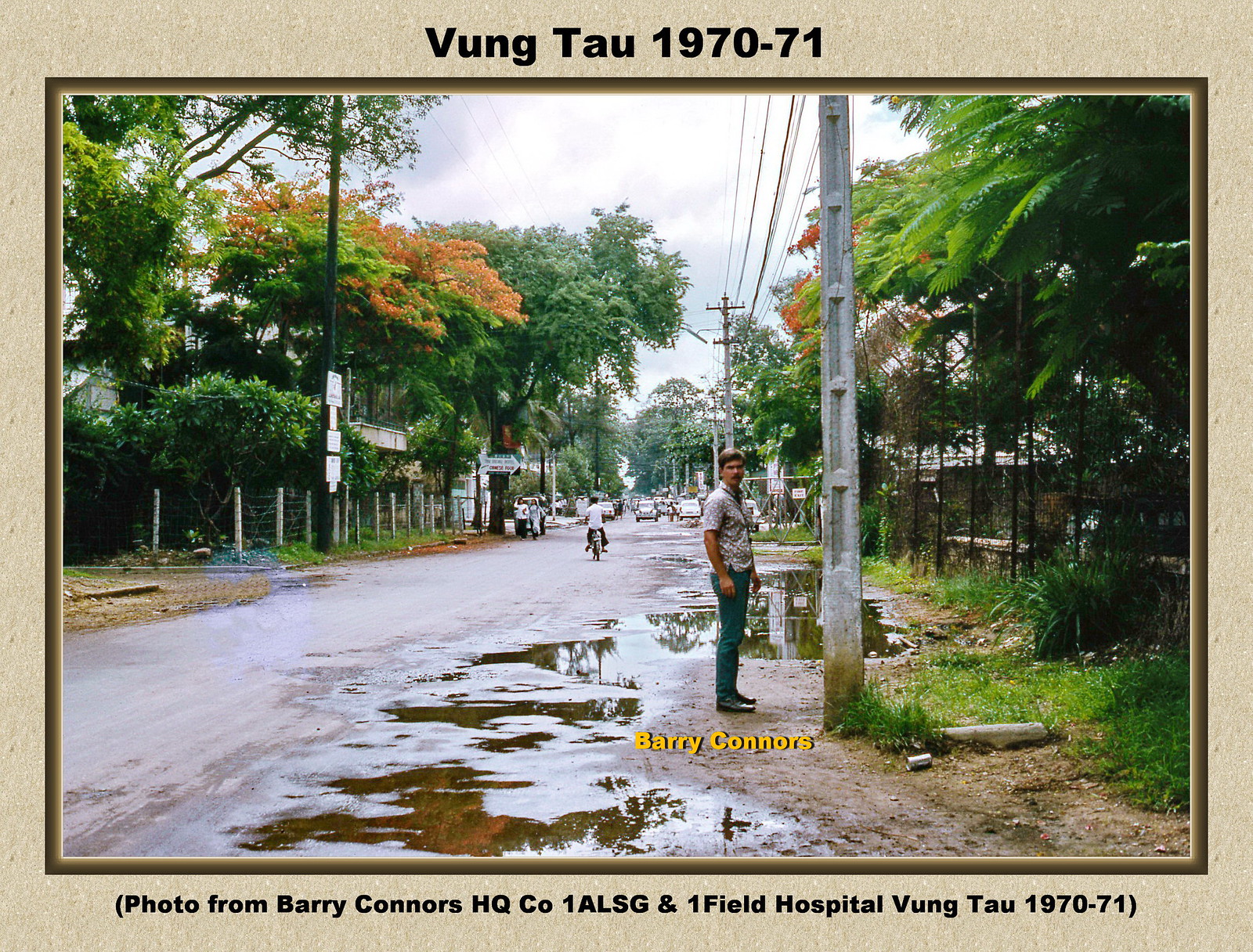The photograph, taken in 1970-1971 in Vung Tau, Vietnam, as indicated by the black text captions at both the top ("Vung Tau 1970 to 71") and bottom ("Photo from Barry Connors HQ CO 1 ALSG and one field hospital Vung Tau 1970 to 71") of the image, depicts a wet, muddy dirt street after a rain, with visible puddles. A white man, identified by the yellow text beneath him as Barry Connors, stands in profile near a pole at the roadside, dressed in a brown shirt, green slacks, and black shoes. The scene captures a mix of local life and military presence: a man on a moped is seen driving away from the camera, while in the distance, there are several cars, palm trees, other trees, women walking, and utility poles, suggesting a neighborhood underdeveloped and in disrepair, lined by lush greenery.